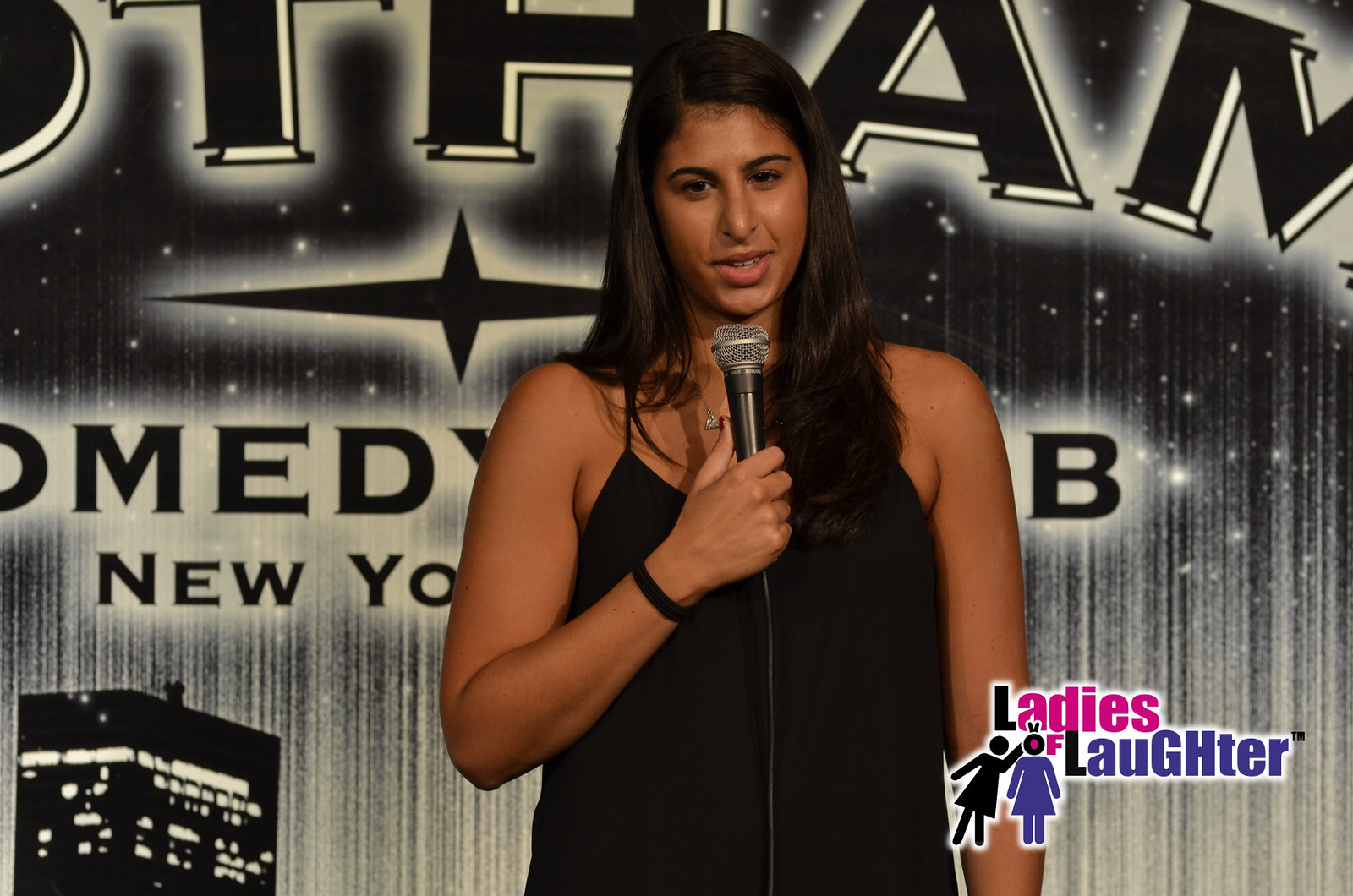The photograph captures a female comedian performing at the Ladies of Laughter event in New York. She is dressed in a strapless or sleeveless black top, accessorized with a silver necklace and a black wristband. Her long brown hair cascades down to her chest, and she holds a microphone with a silver top in her right hand, just below her mouth. She is looking slightly to the bottom left with her mouth partially open, suggesting she is mid-speech or joke. The background features signage from Gotham Comedy Club, partially reading "THAM" and "comedy," set against a black and white backdrop that includes a faded, period-looking card depicting a nighttime cityscape with lights in the windows. The lower part of the background contains some shiny elements reminiscent of stars. In the bottom right corner of the image, there is a logo for Ladies of Laughter: the letters "A-D-I-S" of "Ladies" are in pink, "A-U-G-H-T-E-R" of "Laughter" are in dark blue with "G-H" capitalized, and two icons of women are incorporated into the design.